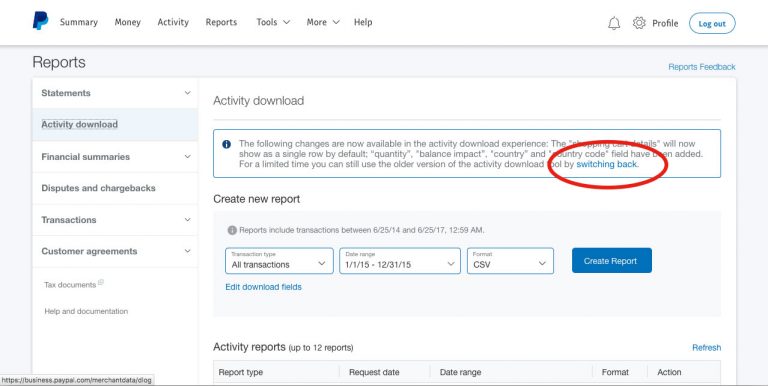The image showcases a portion of the PayPal website interface, specifically capturing the detailed layout of the main Reports screen. Positioned at the top left corner is the PayPal logo, prominently displayed in blue, followed by a series of menu headings: Summary, Money, Activity, Reports, Tools (a pull-down menu), More (a pull-down menu), and Help. To the right-hand side, the interface features a notification bell, a cogwheel settings icon, a profile link, and a logout button, indicating the user is currently logged in.

The user has navigated to the 'Reports' section, and the screen prominently displays several navigation options on the left-hand side, including: Statements, Activity Download, Financial Summaries, Disputes and Chargebacks, Transactions, Customer Agreements, Tax Documents, Help and Documentation. The focus is on the 'Activity Download' option, which has been selected.

On the right-hand side of the screen, under the heading 'Activity Download', there is a blue panel containing text. Notably, a red oval has been drawn around the word "switching" within this panel, emphasizing its significance amidst the otherwise blue text. Below this panel is the 'Create New Report' section, allowing users to specify transaction details, date ranges, and choose the file format for their report. The section culminates in a blue 'Create Report' button situated on the right-hand side, ready for user interaction.